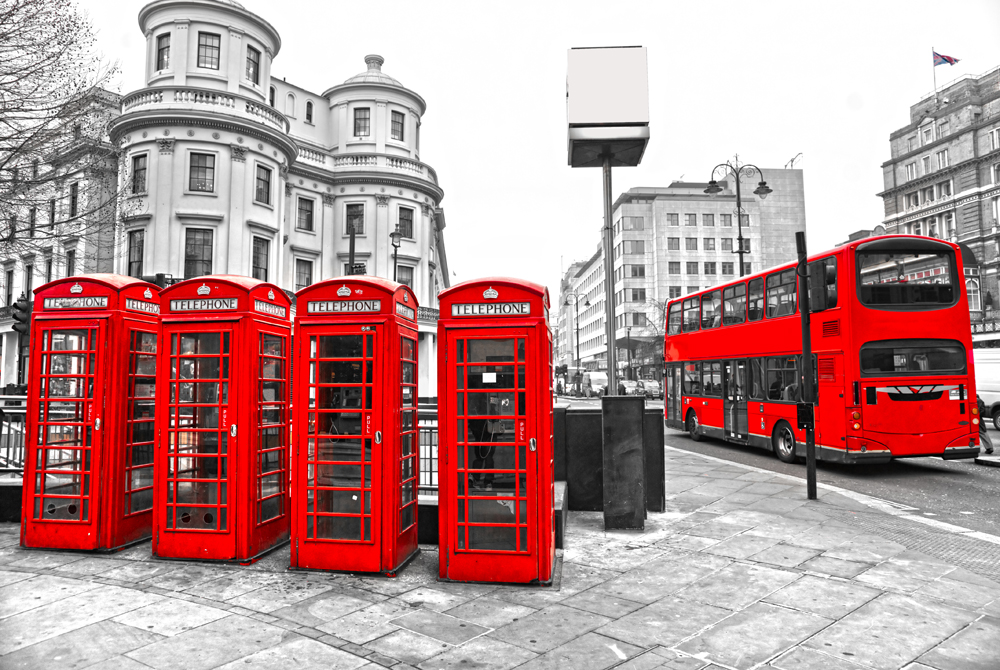This image appears to be a color pop photograph of a historic city scene, likely from London or somewhere else in the UK. The composition is primarily black and white, highlighting the architectural elegance of older, well-constructed buildings made of stone with intricate facades and railings. The streets, paved with stone, guide the viewer's eye to the left side of the photograph where four quintessentially British telephone booths stand in a striking red, each with glass panels framed by the red outline and marked "TELEPHONE" at the top. To the right, a double-decker bus in the same vivid red hue is seen driving away from the viewer, providing a stark contrast against the monochrome surroundings. The positioning of the red telephone booths and the quintessential London bus draws the viewer's attention, standing out as vibrant focal points in this otherwise grayscale cityscape.